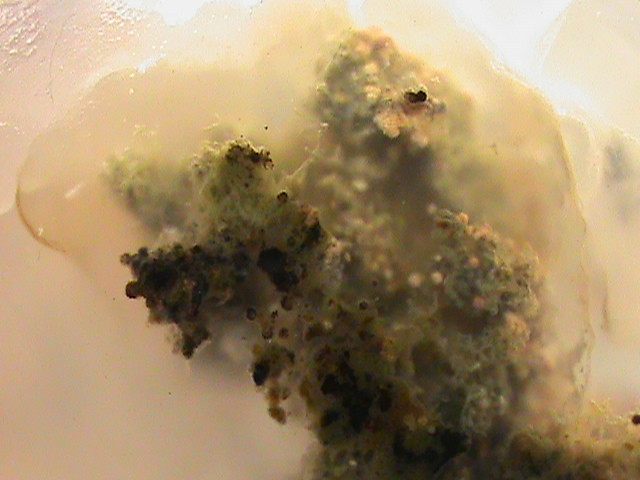The image depicts a detailed, close-up view of a murky, frosted glass or plastic surface immersed in a liquid, possibly water. The glass appears discolored and brownish, indicative of dirty or stained conditions. Growing on and around this surface is a textured, chunky material, possibly a type of fungus, algae, or mold. This growth varies in color from brownish-green to dark nearly black areas where it touches the frosted surface. The photo's background is predominantly white, with reflective qualities at the top that highlight the varying densities and colors of the organic material, which appears thick and almost gelatinous in the center, adding a slight sense of repulsion. The scene bears resemblance to an aquarium wall or a petri dish under scientific study, with the murky, possibly microbial substance thriving in a liquid medium.